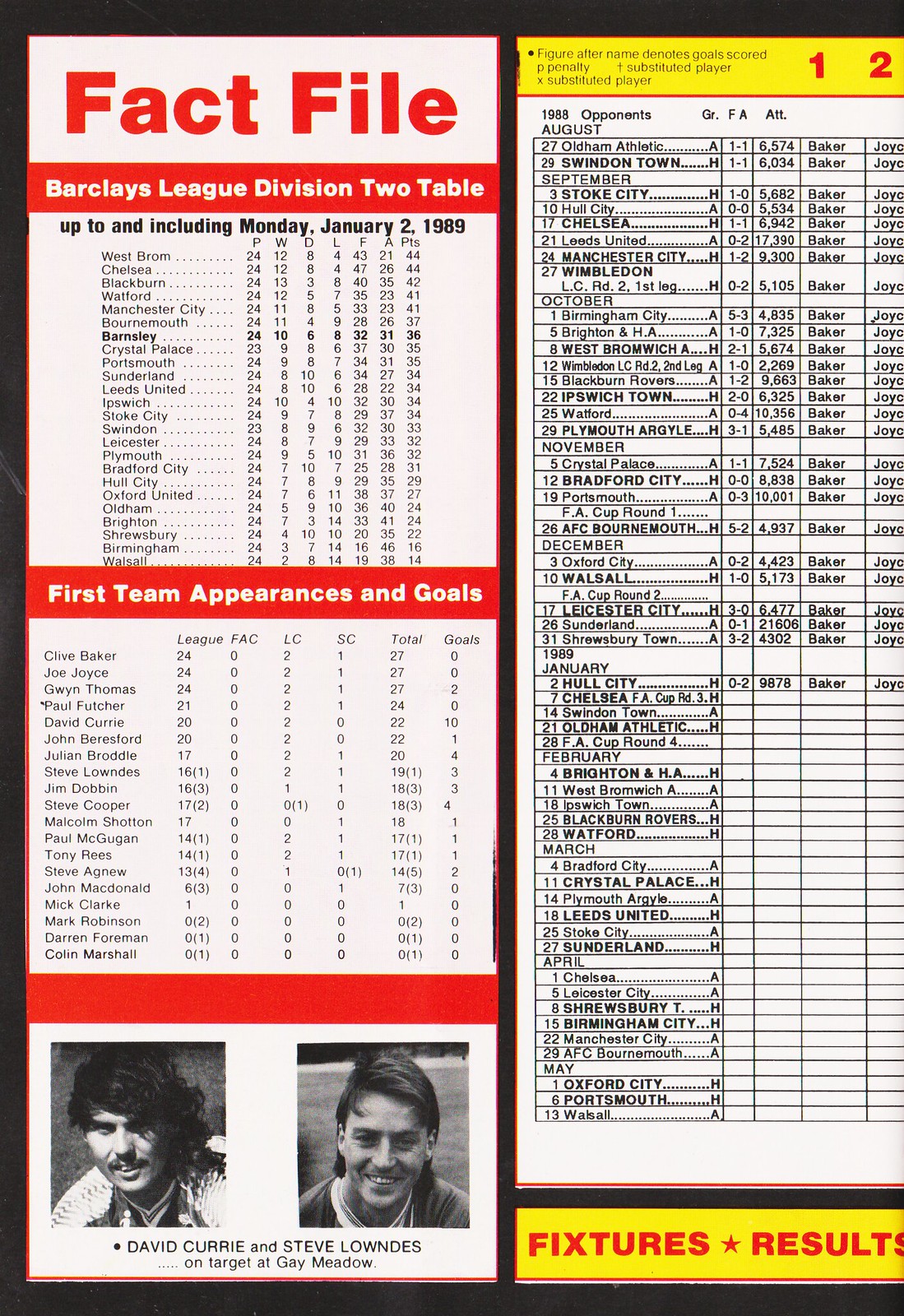The image presents a detailed fact file for the Barclays League Division 2, prominently featuring statistical charts and visuals. On the top left, a red banner showcases the title "Barclays League Division 2 Table," listing all teams in the division along with their respective statistics, including Points, Wins, Draws, Losses, For, Against, and Points Total (PWD LFA PTS). Below this, another red banner labeled "First Team Appearances and Goals" provides individual player statistics, broken down into different competitions such as League, FAC, LC, and SE, and tallying the total goals scored by each player. 

In the bottom left, portraits of two players, David Curry and Steve Lowndes, are featured with the caption "on target at Gay Meadow." The right half of the image is a vertically organized section that includes a list of fixtures and results, with scores from matches played from August 1988 to May of the following year. This section also features match dates, opponents, and outcomes, all written predominantly in red text over a yellow background, with a red star separating columns. The image also notes that it was Friday, March 7th, adding a sense of timestamp to the document.